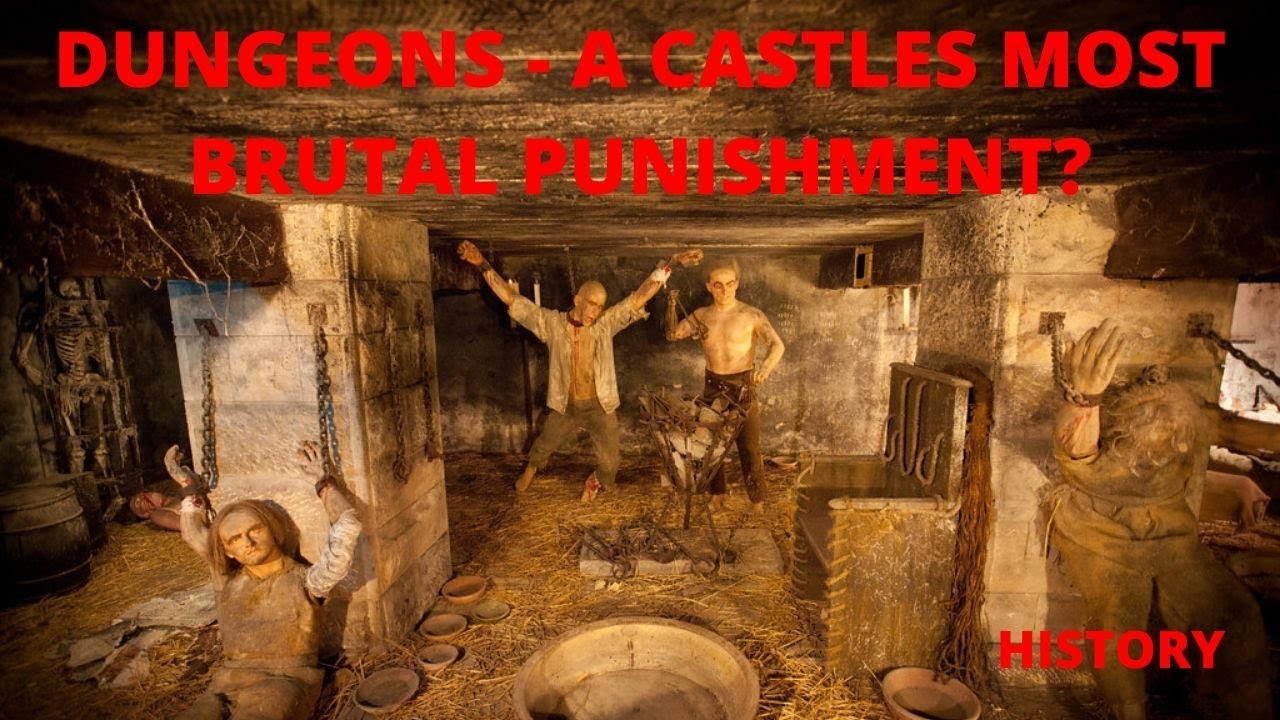This color photograph titled "Dungeons: A Castle's Most Brutal Punishment?" features a detailed museum display of a medieval dungeon. The eerie scene includes several mannequins in various states of torment, evocative of the brutal punishments of the era. 

At the far left of the image stands a skeleton next to a dark barrel, adding to the macabre atmosphere. An expressionless mannequin chained to a pillar looks towards the viewer, his hands bound in manacles as if in despair. In the center, another mannequin hangs from the ceiling by his arms, his body streaked with simulated blood, one foot visibly stained. A bare-chested jailer stands nearby, brandishing an unidentified instrument, suggesting the torment the hanging figure endures.

To the right, another mannequin slouches with its head down, shackled to the dungeon wall. A table stands next to the right pillar, with several bowls scattered across the hay-strewn floor, enhancing the dilapidated, historical aura of the setting. The red text at the top reads, "Dungeons: A Castle's Most Brutal Punishment?" with the word "HISTORY" appearing in the bottom right corner, anchoring the scene in its educational and historical context.